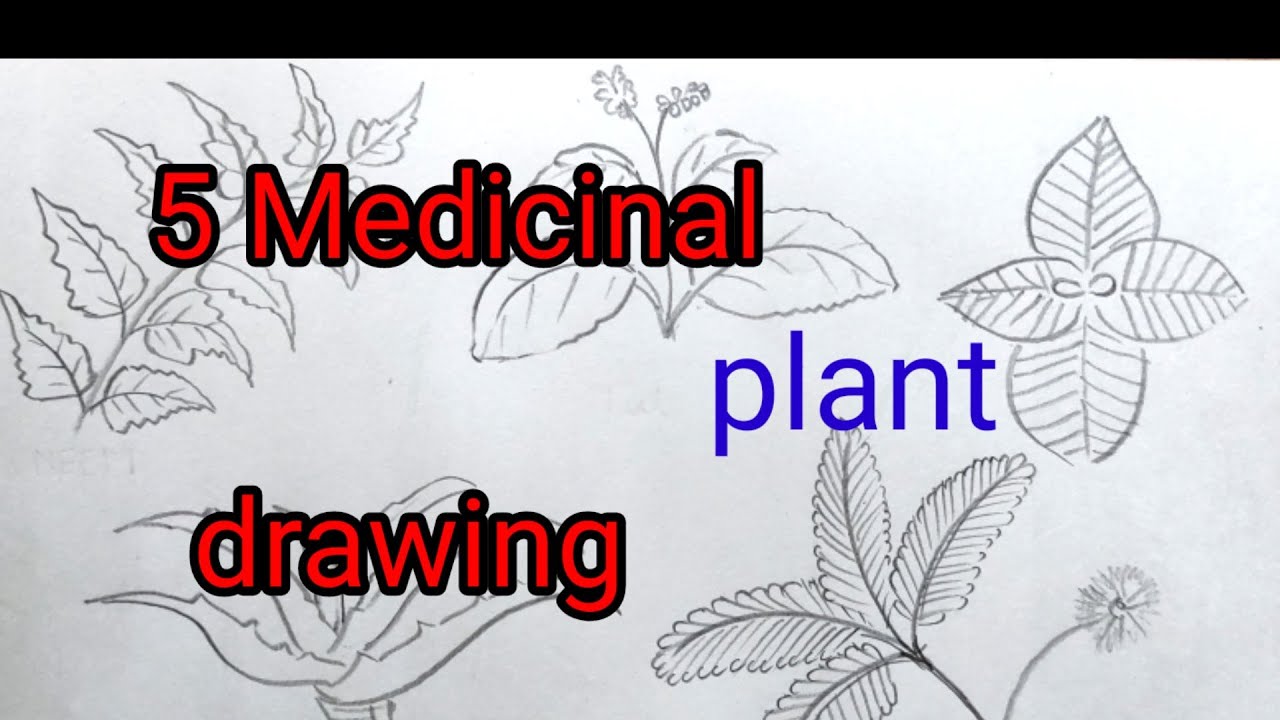This image features a detailed pencil or charcoal drawing on a white background, depicting five different medicinal plants in black and white. Each plant exhibits distinct characteristics such as jagged, pointed leaves and intricate branching stems. The left-most plant shows a stem with several jagged leaves and a singular leaf at the branching tip. Another plant in the center has a vertical stem splitting into branches with small seedlings at the top, flanked by two large leaves at the base and two smaller ones above them. 

Overlaying the illustration is text created in a word processor, reading "Five Medicinal Plant Drawing." The words "Five Medicinal" are in large red lettering with a black border around each letter, while "Plant" is in blue, and "Drawing" is also in red with a black border. A thin black border runs horizontally across the top of the image, enhancing its framing. The overall composition combines artful detailing of the plants with vibrant, attention-grabbing text that categorizes the botanical sketches.